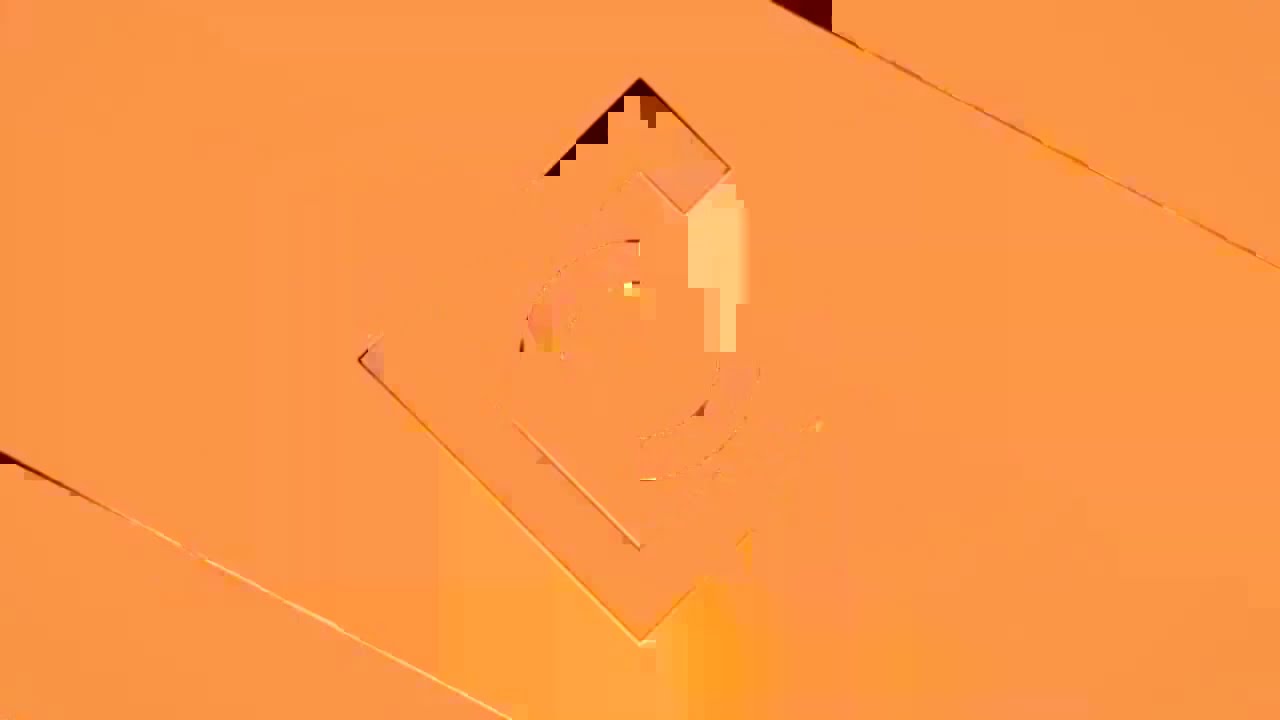The image depicts the interior of a ceiling predominantly painted in an orange hue. However, the ceiling bears evident signs of discoloration, marked by yellowish staining that spreads across several feet, suggesting possible water damage. Distinct cracks run through the image, with prominent ones on the upper right and bottom left corners, resembling angles and triangular formations. Centrally, an angular square cutout is visible, with a section in the top middle revealing blackness behind the surface. The area surrounding this square also displays varied shades of yellow-orange, particularly at the bottom, enhancing the impression of material fatigue or damage. The image's texture appears pixelated, adding to the complexity of the scene.